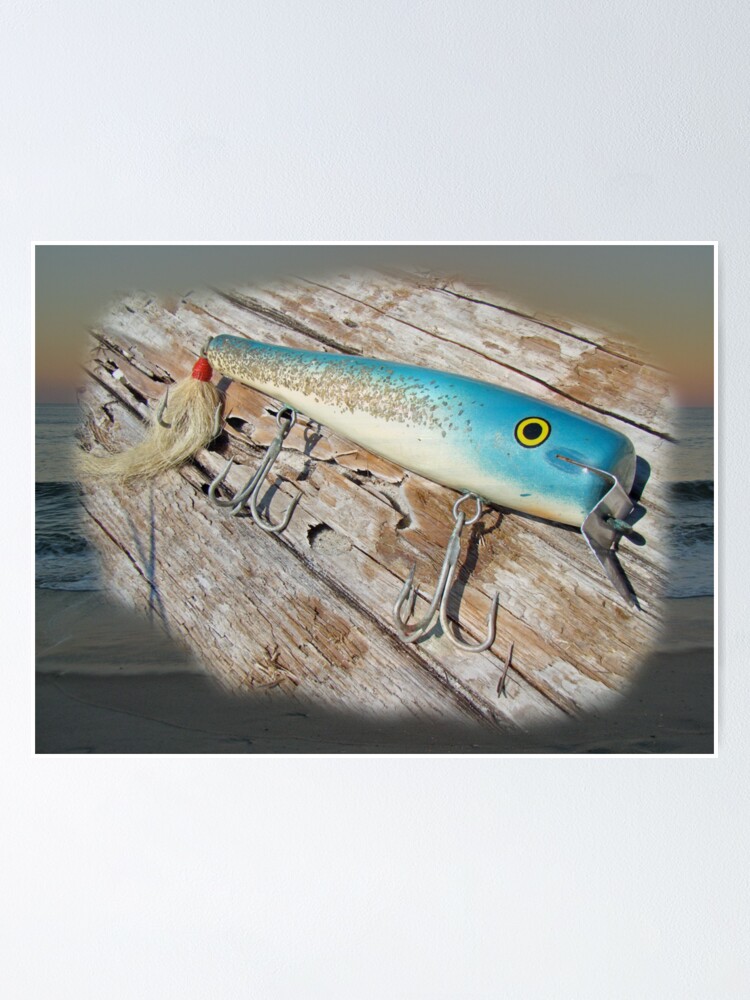The image displays an intricate photograph of a vintage fishing lure, prominently centered against a textured, weathered wooden board. The lure is shaped like a fish with a vivid teal-blue body, a white underside, and striking yellow eyes with black pupils. The fish's intricate design includes a tail adorned with red feathery appendages and two shiny silver hooks hanging along its body. The fishing lure's mouth area features a metallic attachment for linking to a fishing line. This detailed photograph is inset within an antique-style frame, positioned in the middle of a tall white rectangular background, casting a subtle shadow. Fading in the background, there's a serene ocean sunset scene, blending seamlessly with the main focal point, enhancing the nostalgic and tranquil essence of the image.